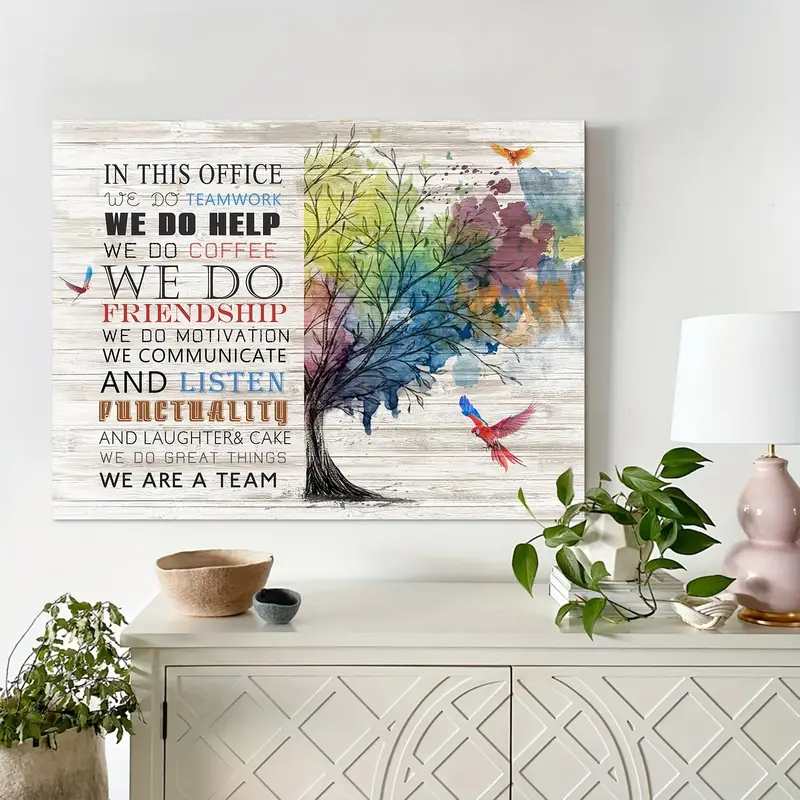A white wall serves as the backdrop for a carefully arranged scene that features a sleek, white entertainment cabinet, designed with a trellis-like texture and rounded insets, of which only the top half is visible. To the left, the corner of a pot containing a lush green plant peeks into view. Atop the cabinet, there’s a light brown bowl, a small dark gray bowl, a pot with vibrant green leaves which appears to be placed on top of a book, and some other small decorative items. On the far right of the scene stands a pink-based lamp with a white shade. Above the setup, a wide horizontal print is prominently displayed. The print, which seems to be an artwork advertised for sale potentially on websites like Amazon or Wayfair, illustrates a tree with blue and red hues, complemented by a collection of colorful parrots. Superimposed on the left side of the image are inspiring words: "In this office, we do teamwork, we do help, we do coffee, we do friendship, we do motivation, we communicate and listen, punctuality, laughter, and cake, we do great things, we are a team." The artwork appears to be mimicking the look of gray wooden boards laid out horizontally, forming a striking and motivational centerpiece above the cabinet.